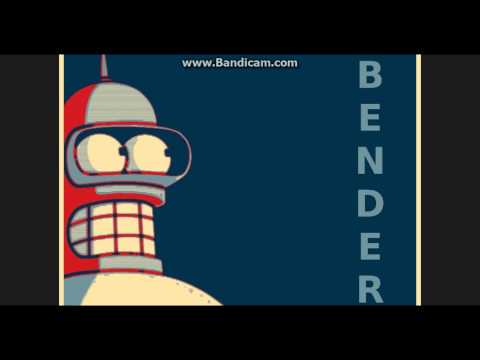The image depicts a cartoon rendering of Bender, the robot character from the show "Futurama." Positioned on the far left, Bender has a dome-shaped head, large expressive eyes, and an open mouth showcasing approximately 12 teeth, displaying an expression of concern or interest. The background is a dark blue with thin white borders on the left and right sides. Vertically aligned on the right in light blue letters is the word "Bender." A reddish tint accents Bender’s otherwise gray robotic exterior. The website URL "www.bandicam.com" is prominently displayed in white text at the very top of the image, suggesting it serves as an advertisement for Bandicam.